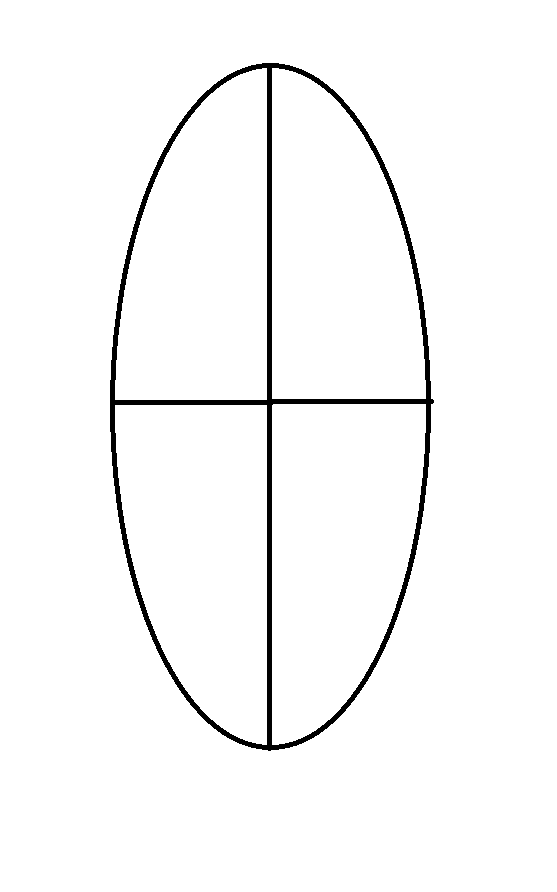The image features a vertically oriented oval with a plain white background. Dominating the image is the elongated oval that is taller than it is wide, resembling a stretched-out egg but with symmetrical ends. This oval is divided into four equal sections by two straight black lines that intersect perpendicularly in the center, forming four right angles. Notably, the horizontal line extends slightly beyond the oval's right edge. The simple black-and-white color scheme and the geometric precision give the image a minimalist and almost technical feel, reminiscent of a preliminary sketch for a face, where the circle and T-lines help guide the placement of facial features.